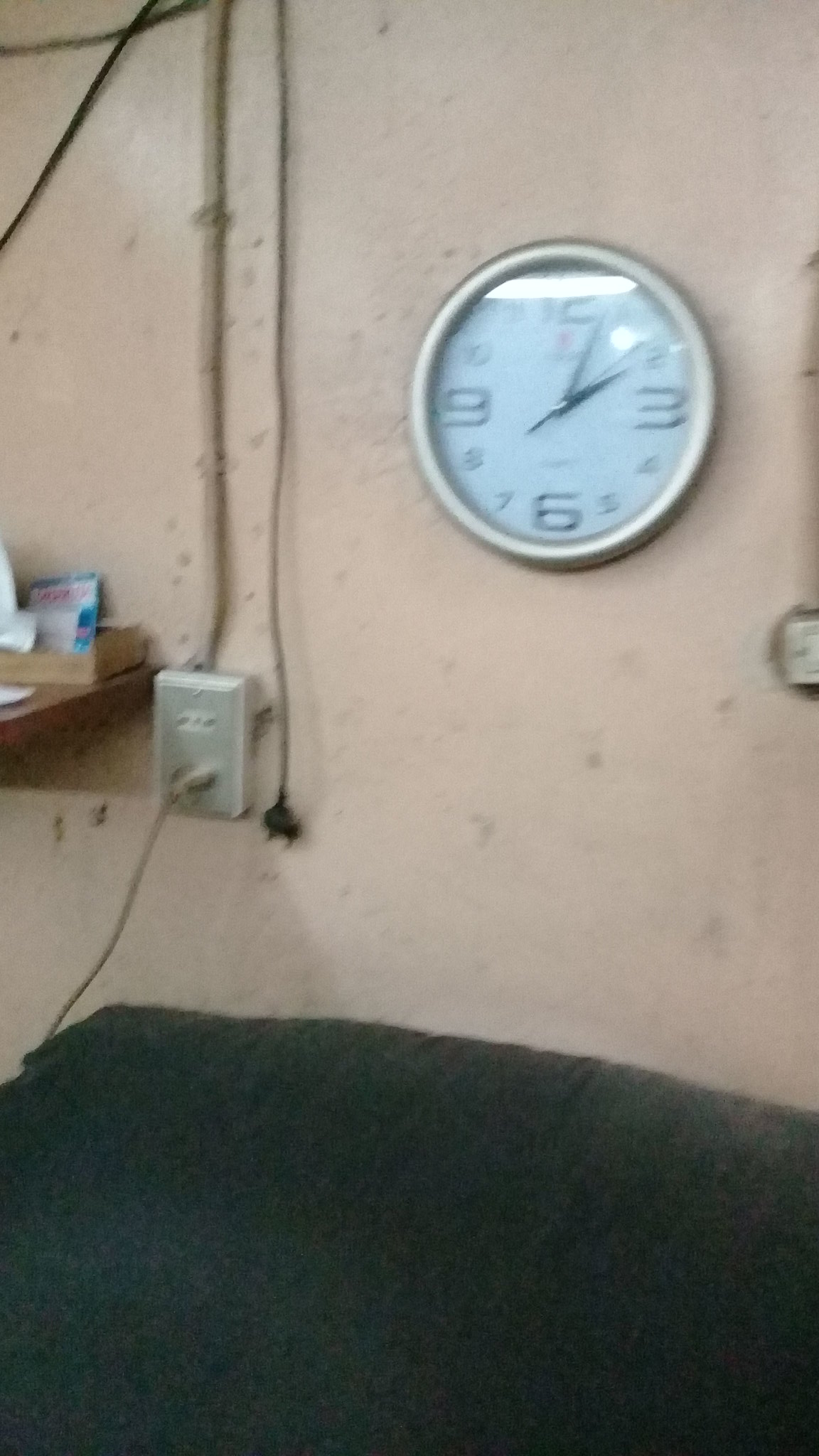The rectangular photograph, oriented vertically, captures a scene featuring a noticeably dirty beige wall. The image quality is somewhat blurry and of poor resolution. In the upper right corner of the wall, a silver wall clock with a white face is mounted. The clock prominently displays the numbers 12, 3, 6, and 9 in black, alongside black hour and minute hands indicating the time as 2:05. Below the clock, there is a black object—possibly a dark table—pushed against the wall. Additionally, a protruding electrical outlet is visible to the lower left of the clock, from which a beige cord is trailing out.